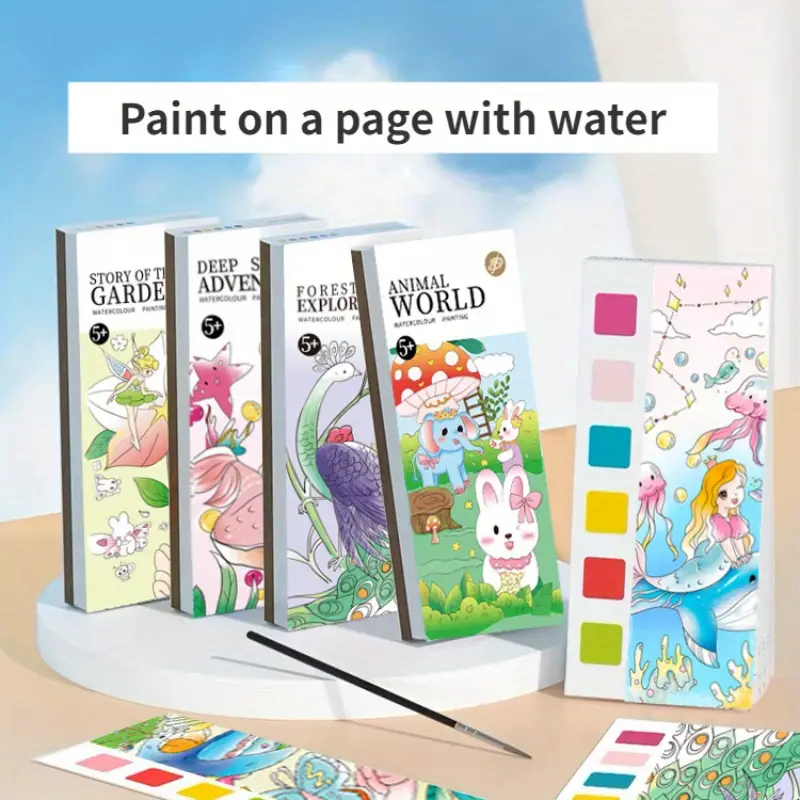The image features an assortment of children's watercolor painting books set on a white flat pedestal, and an open book showing squares of watercolors designed for use with the books. Vibrant colors including pink, purple, blue, yellow, red, and green are visible. Each book is labeled with different themes: Animal World, Forest Explorers, Deep Sea Adventures, and Story of the Gardens, with part of the text slightly obscured but still recognizable. An additional closed book rests beside them. A paintbrush is included, designed to be dipped in water to activate the colors and paint the page. The books are intended for children aged 5 and up, as indicated by the "5+" age label. In the background, you can see a light sky with clouds suggesting a curtain. The books offer a mess-free way for children to enjoy painting, simply requiring water and the included paintbrush.